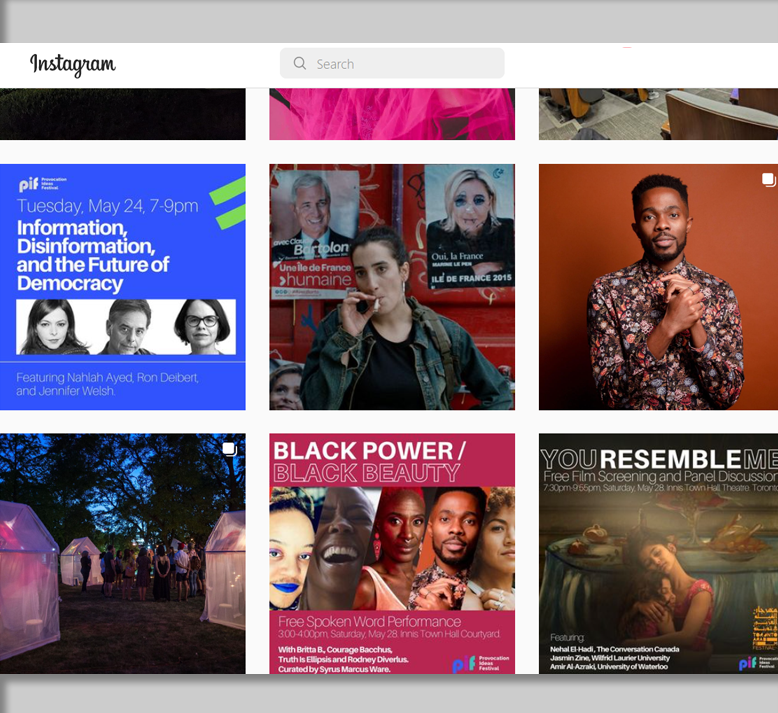This screenshot captures the Instagram interface displayed on a website, characterized by distinctive gray bars at the top and bottom of the screen. The interface itself features a white header bar with "Instagram" elegantly written in black cursive font, positioned in the left corner. Central to this header is a gray search field adorned with a magnifying glass icon, prompting users to "Search" in gray text.

Beneath the header, the content is organized into two rows consisting of three square thumbnails each. The first thumbnail in the top-left corner is notable for its blue background and white text. It announces an event titled "Tuesday, May 24th, 7 to 9 p.m. - Information, Disinformation, and the Future of Democracy."

Directly below this event notice, there is a white rectangular image featuring the heads of three individuals of Caucasian descent. The trio includes, from left to right, a young brunette woman, an older man, and another brunette woman adorned with glasses.

Adjacent to this rectangle, the second square image showcases a white woman smoking a cigarette against a vividly graffitied red wall. This woman has brown hair and eyes, and she is dressed casually in a black shirt layered with a jean jacket.